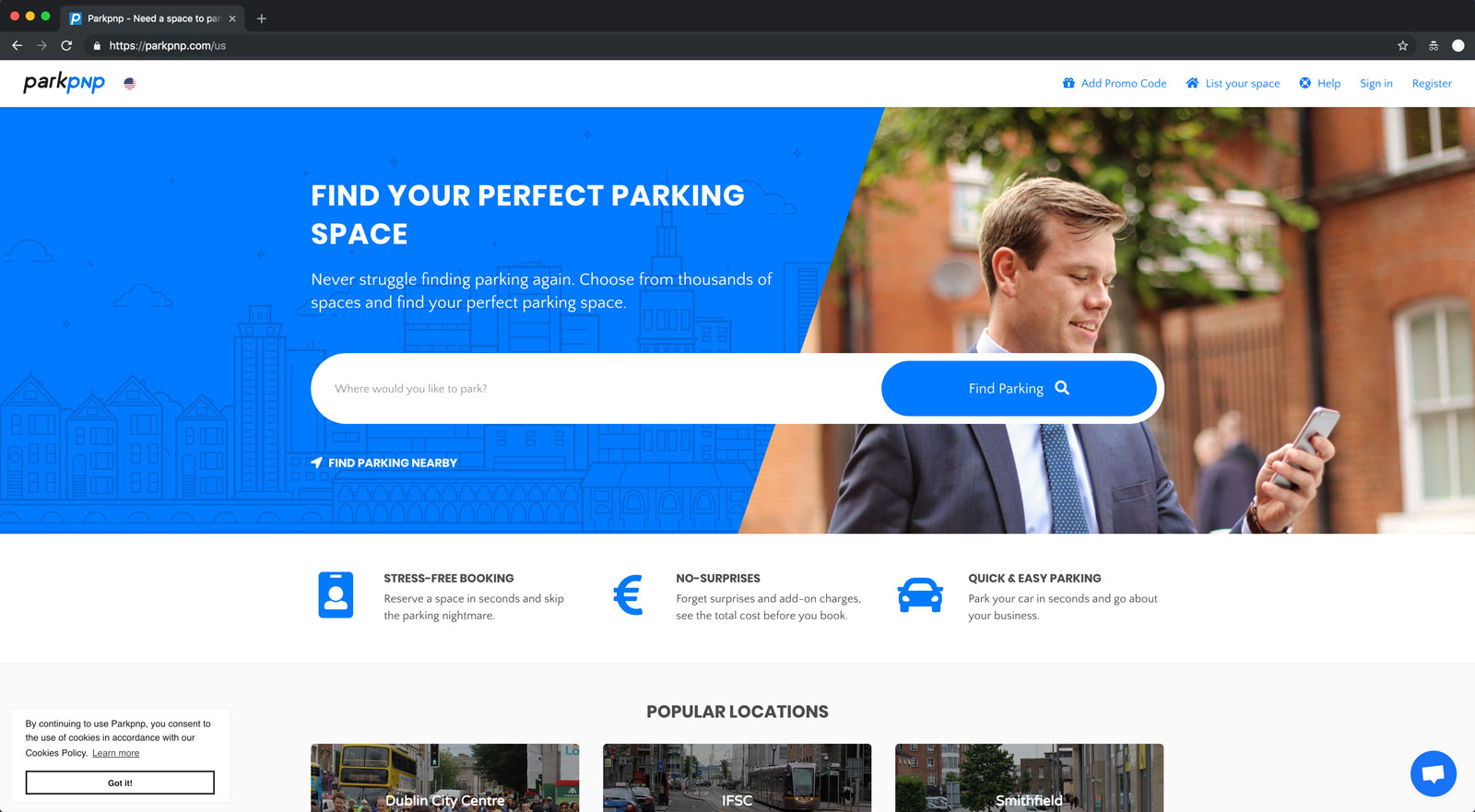A detailed and cleaned-up caption for the image could be:

"A screenshot of a website offering convenient parking solutions is prominently displayed. The website promises a stress-free booking experience, allowing users to choose from thousands of parking spaces to find their perfect spot. The header reads, 'Find Your Perfect Parking Space' and emphasizes easy, surprise-free booking. The site features a blue section with a city skyline silhouette and highlights popular parking locations.

In the forefront of the image is John, engrossed in his smartphone. He stands in front of a red brick building that has several windows and a few visible gates. The surrounding environment suggests a pleasant day, as the trees in the background still retain their leaves. On the side of the screenshot, there's a small square area named 'Park,' which appears to be pretty empty."